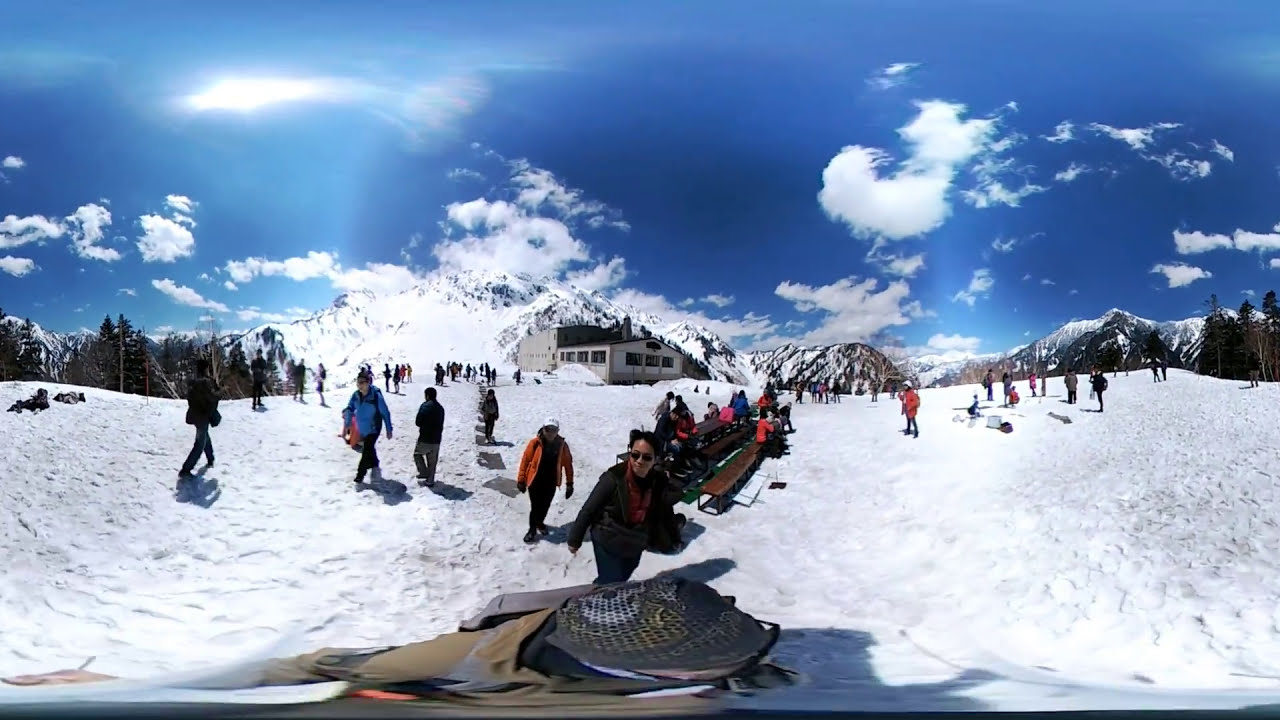The image depicts a lively ski resort enveloped in a pristine white snowy landscape. In the central background, a white building structure, possibly a lodge where visitors can check-in and warm up, stands out. Majestic, snow-capped mountain ranges stretch across the horizon, with a vibrant blue sky adorned by a few wispy clouds. Scattered around the scene are various people, all clad in heavy winter gear including jackets, boots, hats, and sunglasses to shield against the bright sun. These individuals appear to be engaged in or prepared for a range of winter activities such as skiing, snowboarding, and sledding. A picnic table with attached benches occupies the center of the picture, where some people are seated, while others move towards the camera, suggesting a friendly and relaxed atmosphere. On the far edges of the image, children are seen sledding. The bottom of the screen features a person taking a selfie, capturing the joyful ambiance of the moment. The entire scene portrays a bustling, cheerful vibe of people enjoying a wintery day amidst breathtaking natural beauty.